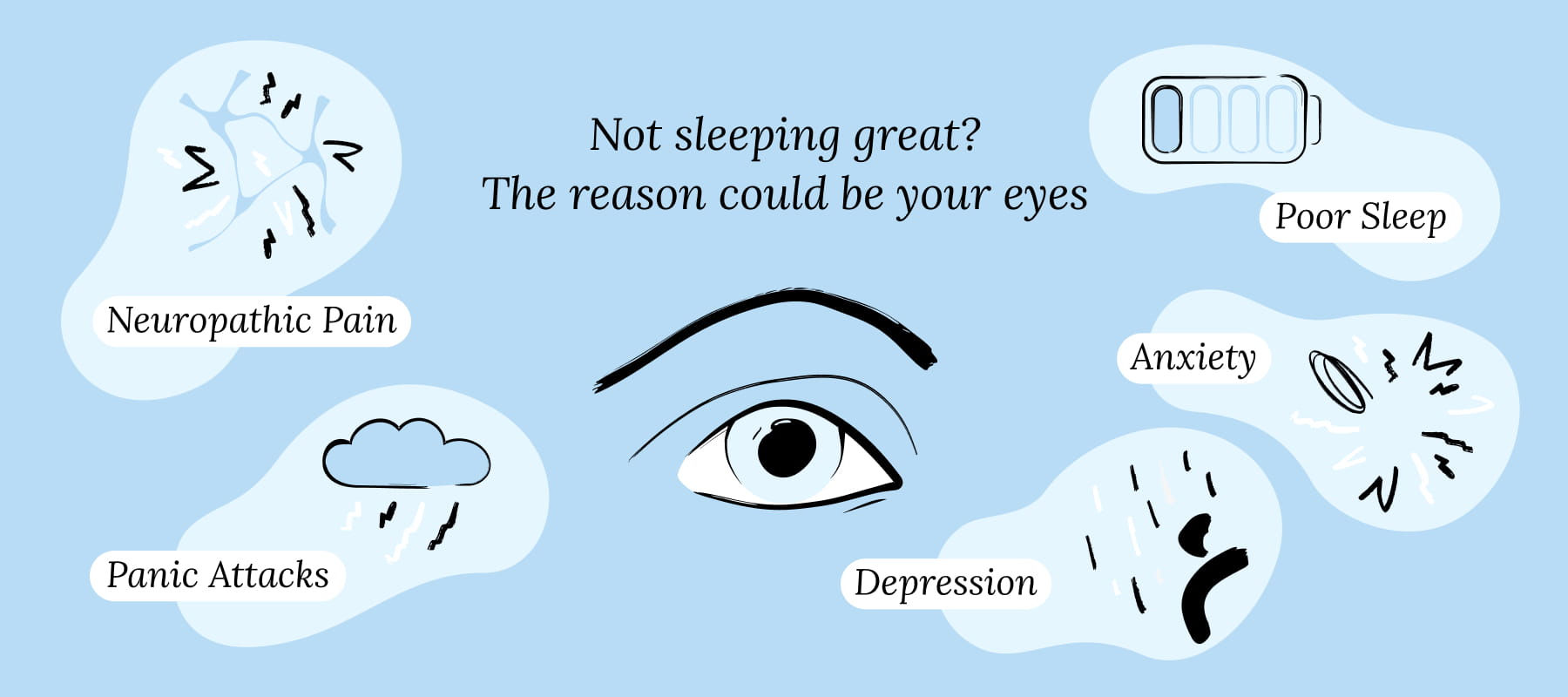This image is an informational poster about the dangers of poor sleep, set on a light blue background. At the top center, bold black text reads, "Not sleeping great? The reason could be your eyes." Beneath this, a simplistic illustration of an eye with a black eyebrow above it is prominently placed. To the left, two light blue bubbles convey potential consequences of poor sleep: the first contains abstract lines labeled "Neuropathic Pain," and the second features a thundercloud with lightning bolts labeled "Panic Attacks." On the top right, another bubble displays a bed with the label "Poor Sleep." Below this, a bubble filled with squiggly lines is marked "Anxiety," and the bottom bubble shows an upside-down smile surrounded by raindrops and is labeled "Depression." The poster uses crude line art and might be an early draft or the work of a design student. Despite its simplicity, the graphics effectively communicate the negative impacts of poor sleep.